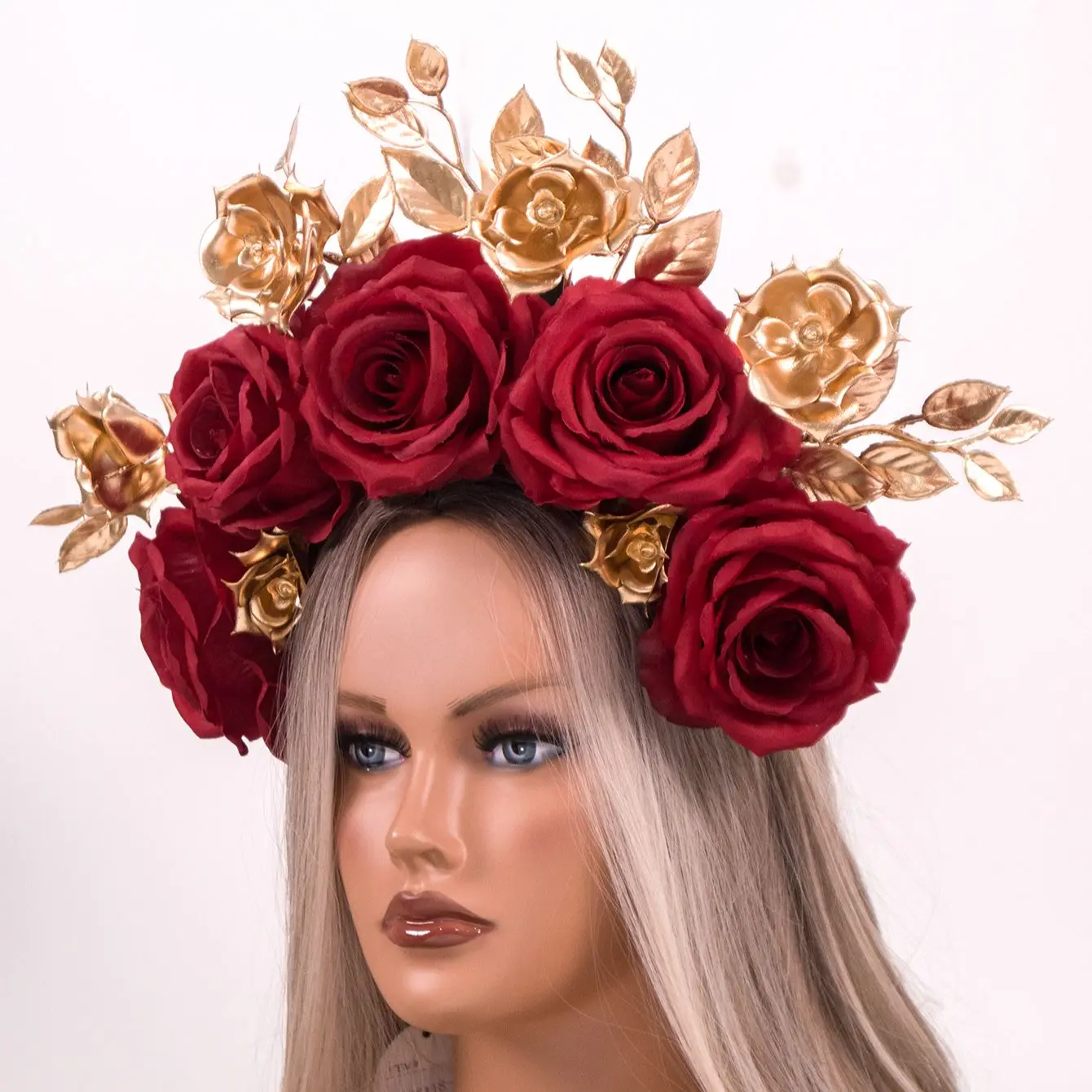This commercial photo, intended for an online shop selling headpieces, features a mannequin head prominently centered and tilted at a 45-degree angle, looking away from the camera. The mannequin has striking blue eyes, framed by long fake eyelashes, reddish eyeshadow, glossy lips, and painted eyebrows, adding to her lifelike appearance. She sports a blonde wig. Atop her head rests an ornate rose headdress, designed in a flower crown style. The headdress is adorned with five soft fabric red roses and six metallic-looking gold roses. The red roses provide a lush contrast to the gold roses, which come with metallic golden leaves that might be crafted from malleable aluminum for ease of arrangement. Additionally, some gold roses have visible thorns. The overall scene is set against a clean, white background, ensuring the vibrant colors and intricate details of the headpiece stand out.